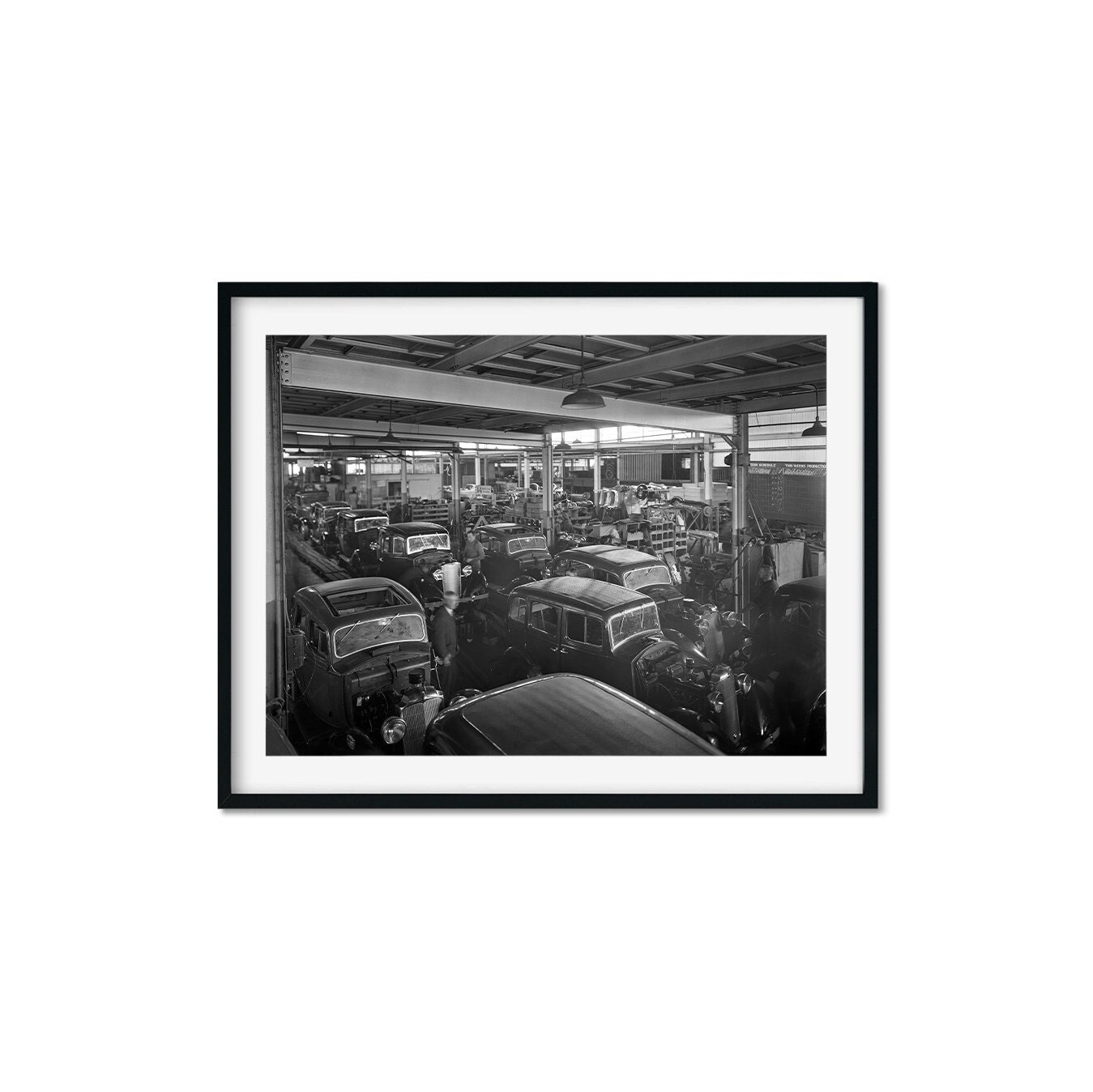This is a detailed black-and-white photograph, framed in a narrow white mat with a thin black edge, depicting an auto factory, likely from the 1940s or 1950s. The factory floor is filled with partially assembled old-fashioned cars, characterized by long hoods and large driver and passenger compartments. The assembly line, appearing automatic, runs through the image, with workers busily installing components as the cars move along. Some workers are slightly blurred due to the motion, indicating the hustle and bustle of the manufacturing process. The factory's ceiling has rafters with single, non-fluorescent light bulbs providing dim lighting, contrasting with some large windows at the back that reveal daylight outside. This snapshot captures a moment in industrial history, emphasizing the labor-intensive work that contributed to the production of these classic automobiles.